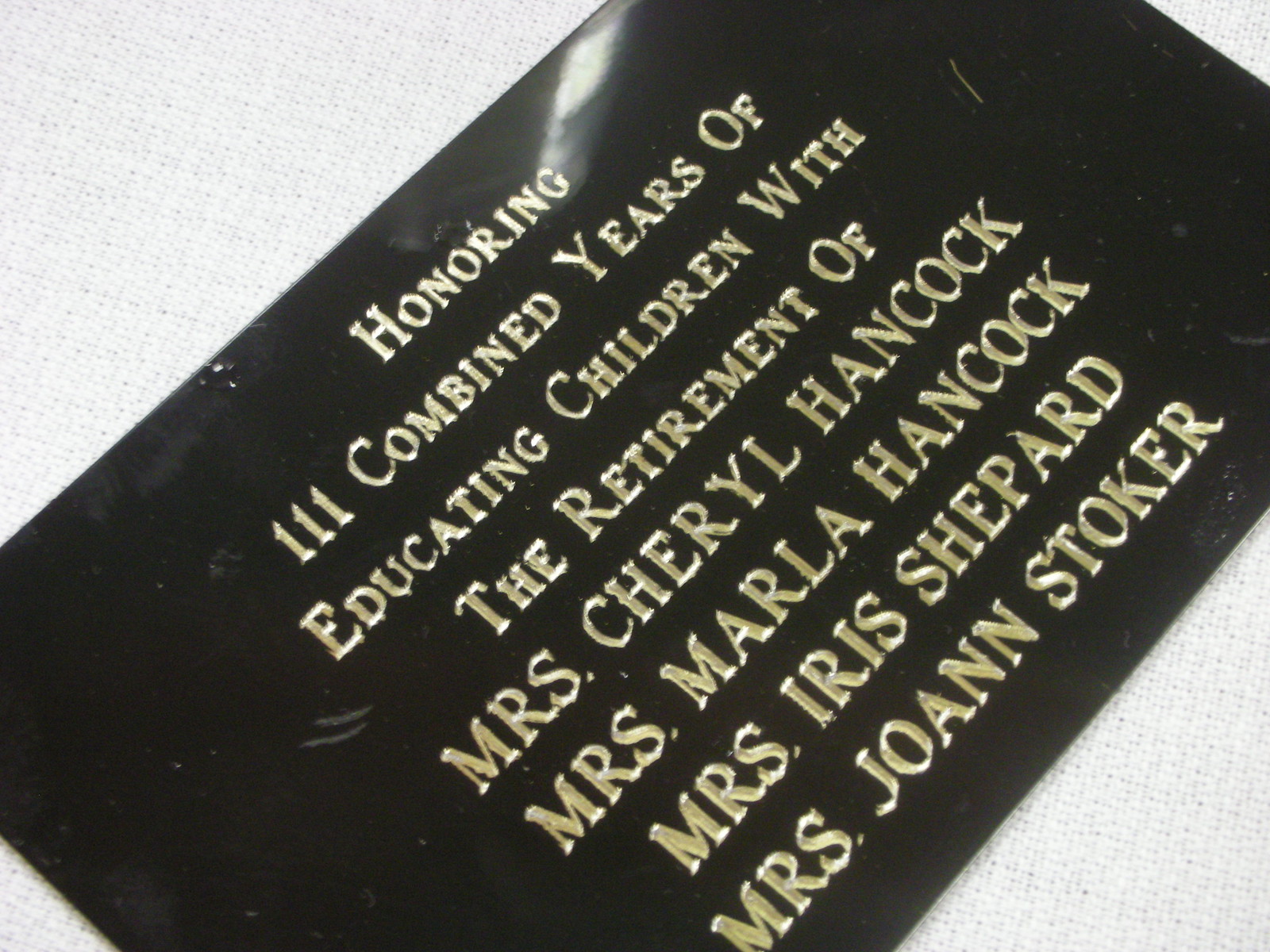The image showcases a rectangular plaque made of a shiny black material, elegantly displayed against a white backdrop. The text, engraved in light gold and fully capitalized, reads: "HONORING 111 COMBINED YEARS OF EDUCATING CHILDREN WITH THE RETIREMENT OF," followed by the names of the four honored educators: Mrs. Cheryl Hancock, Mrs. Marla Hancock, Mrs. Iris Shepard, and Mrs. Joanne Stoker. The names are presented in a slightly larger font than the rest of the text, emphasizing their importance. The plaque, with its dignified appearance, celebrates the distinguished careers of these teachers who collectively devoted 111 years to educating children.